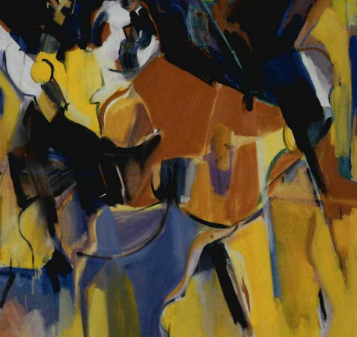This image is a small, square canvas painting rendered in an abstract style. The composition features a chaotic, yet intriguing mix of colors and shapes that draws the viewer in. Key colors in the painting include bold splashes of yellow, black, blue, white, and shades of orange and brown. In the upper left corner, there's a striking swash of black paint, beneath which are splotches of white, yellow, and tan, forming a seemingly random yet compelling pattern. The upper right corner, dominated by dark blue and black lines, also contains touches of red, yellow, and white. The central area features an intriguing blend of orangish-brown hues.

The lower left corner is primarily bluish, accented with strokes of yellow and gray, while the lower right corner showcases yellowish-gold and gray tones. The overall feel is notably abstract, with no clear depiction of any specific object. Nonetheless, the interplay of colors and lines suggests deeper, possibly hidden meanings, inviting viewers to spend time contemplating its possible interpretations. The blend of elements gives the painting a dynamic and vibrant character, characteristic of abstract expressionism.